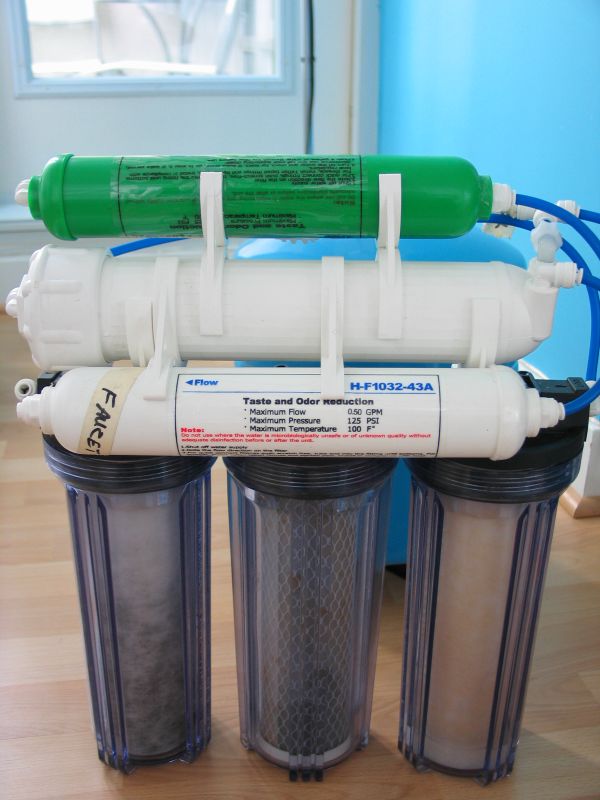This photo depicts a complex home filtration system situated in front of a white doorway. The system consists of three cylindrical canisters stacked vertically, with two larger white ones at the bottom and a green one on top. Each canister is supported by three vertically arranged clear cylinders with black lids, resembling clear drinking cups. Blue tubes connect the top canister to the clear cylinders below. The bottom white canister has text indicating it is for "faucet" and mentions "taste and odor reduction," along with maximum flow, pressure, and temperature specifications. The middle white canister is plain, featuring some ribbing, while the green top canister has print upside down. These components, likely part of a filtration system, rest on a pine-colored wood floor with a turquoise wall in the background. The clear cylinders appear to contain different filter elements, with the left having a cottony material, the middle one containing mesh, and the right one looking empty.